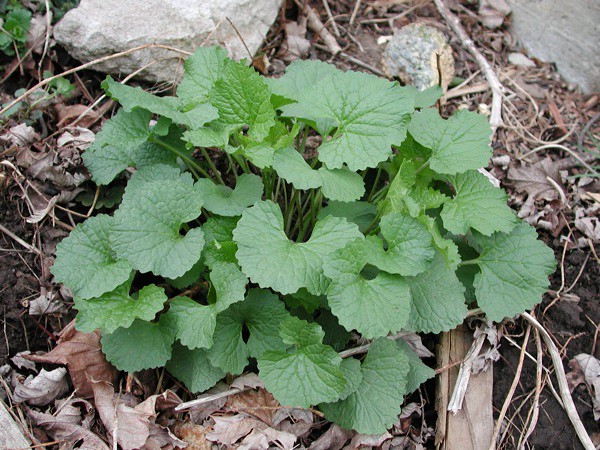The image depicts a dense cluster of Creeping Charlie, characterized by its deep green, heart-shaped leaves, growing amidst a mix of dead, brown, and dried leaves and twigs. Dominating the center of the photo, the Creeping Charlie stands out vividly against the earth-toned backdrop of a brown, mulchy ground scattered with dry grass shoots. A light gray, rigid stone, the largest and most prominent rock in the image, lies towards the top, with additional smaller rocks in the upper right corner. The scene, brightly lit by daytime sunlight, situates the Creeping Charlie along what appears to be the foundation of a wall, glimpsed in the upper right corner. The overall composition, adorned with twigs, dried leaves, and occasional rocks, presents an outdoor setting where nature perseveres despite the barren conditions.